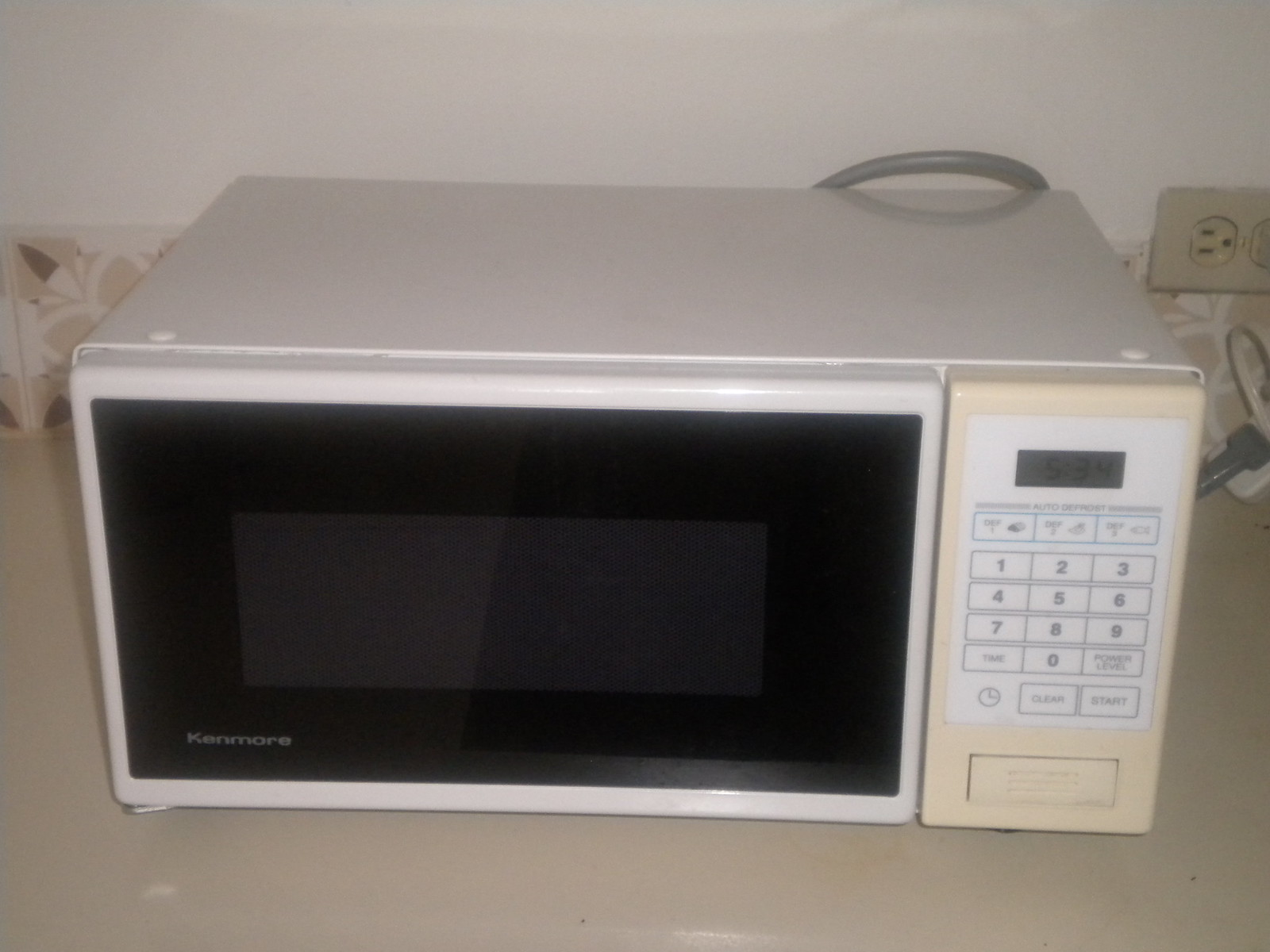The image depicts a white Kenmore microwave resting on an off-white or beige counter. The microwave features a black tempered glass front door, and all the control buttons are white, including the numbers 1 through 9 and 0, the clear and start buttons, and an off-white button to open the door. The digital timer on the panel shows 34 seconds. To the right of the microwave, there's a gray cord leading to a beige outlet and plug. The background includes a white wall and an off-white tile partially visible behind the left portion of the microwave. Additionally, a flowery wallpaper border with neutral colors is located on the lower half of the left wall. The microwave appears slightly dirty, indicating it has been used.